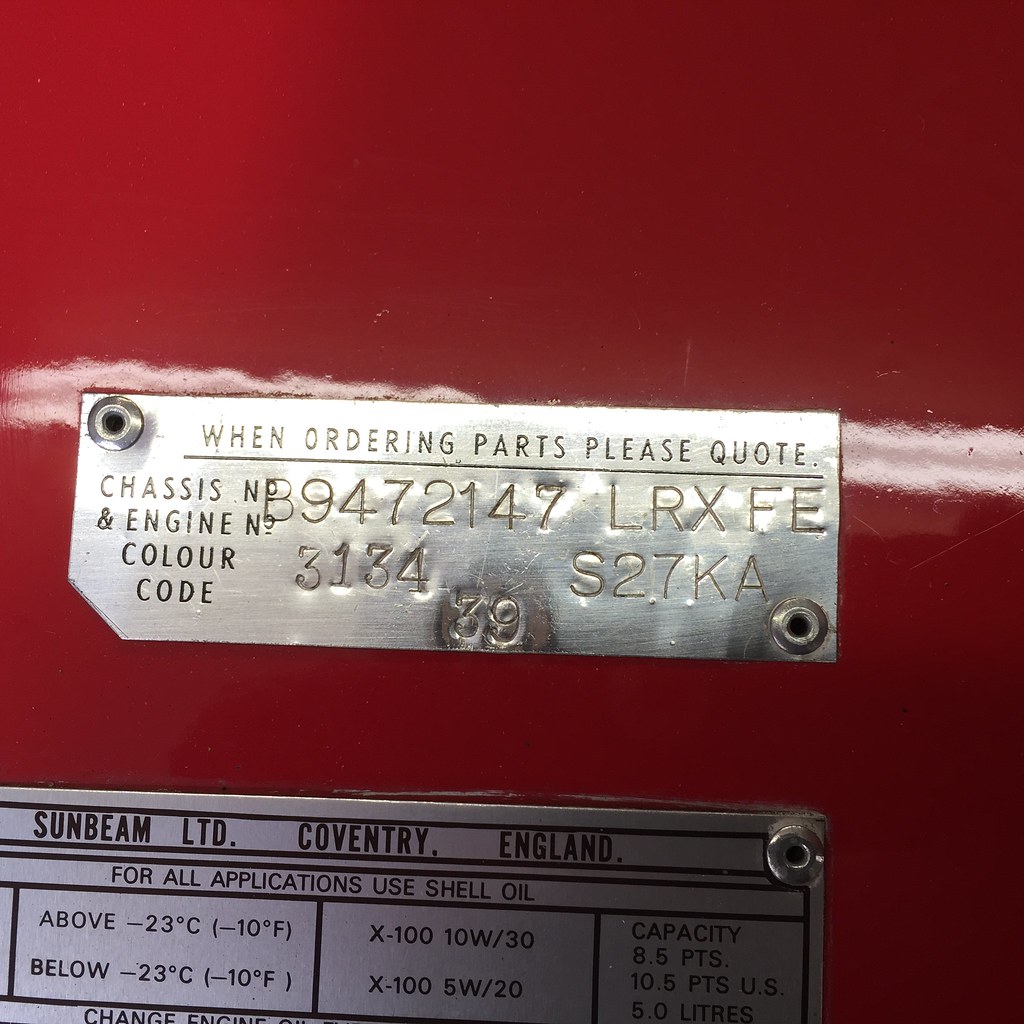The image showcases two metal plaques mounted on a shiny, red, metallic surface, likely indicating a vehicle component from Sunbeam Limited, Coventry, England. The upper plaque, bolted at the upper left and lower right corners, contains critical identification information, including the chassis number "B9472147LRXFE," and the engine number "3134S27KA," along with a color code "39." Additionally, it directs the use of this information when ordering parts. A lower plaque displays operational details, specifying the use of Shell oil for all applications and providing precise operating temperature ranges: "above -23°C (10°F)" and "below 10°C (50°F)." It also outlines oil viscosity requirements "10W-30" and "5W-20," and mentions oil capacities "8.5 PTS, 10.5 PTS US, and 5.0 liters." The meticulous arrangement of the plaques, with their reflective and bolted placement on the red surface, underscores the importance of these technical details.